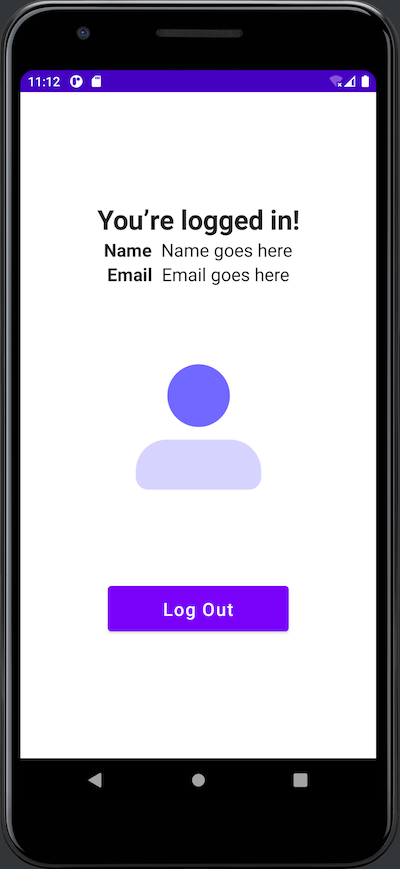The image showcases a mobile device, likely a smartphone or tablet, identifiable by its rectangular, rounded exterior border. Prominently on the top bezel, there's a grid-like area signifying a speaker or microphone, along with a front-facing camera positioned towards the left. 

A thin violet header at the top of the screen displays the time, "11:12," towards the left. Adjacent to it, on the right side of the header, is a white circle featuring a purple "R" within it. Next to this circle, there is an icon representing a SIM or memory card, which is white in color. Moving further to the right, the Wi-Fi symbol is visible, though it shows no connection. To its right, the data signal icon indicates four out of five bars of connectivity, followed by a fully charged battery icon.

Below the header, the main content begins with a light gray background bearing bold black text that reads, "You’re logged in!" 

Following this:
- The word "Name" is in bold, with "Name goes here" in regular font beneath it.
- The word "Email" is in bold, followed by "Email goes here" in regular font.
- An icon resembling a user silhouette is present, comprised of a medium violet circle representing the head and a light purple oval, squared off at the ends, symbolizing the upper body.

Beneath the user icon, there is a violet-colored rectangular button labelled "Log out" in white text.

At the bottom of the screen, traditional Android navigation buttons are visible:
- A gray arrowhead pointing to the left acts as the back button.
- A circle in the middle represents the home button.
- A square on the right signifies the windows or tabs option.